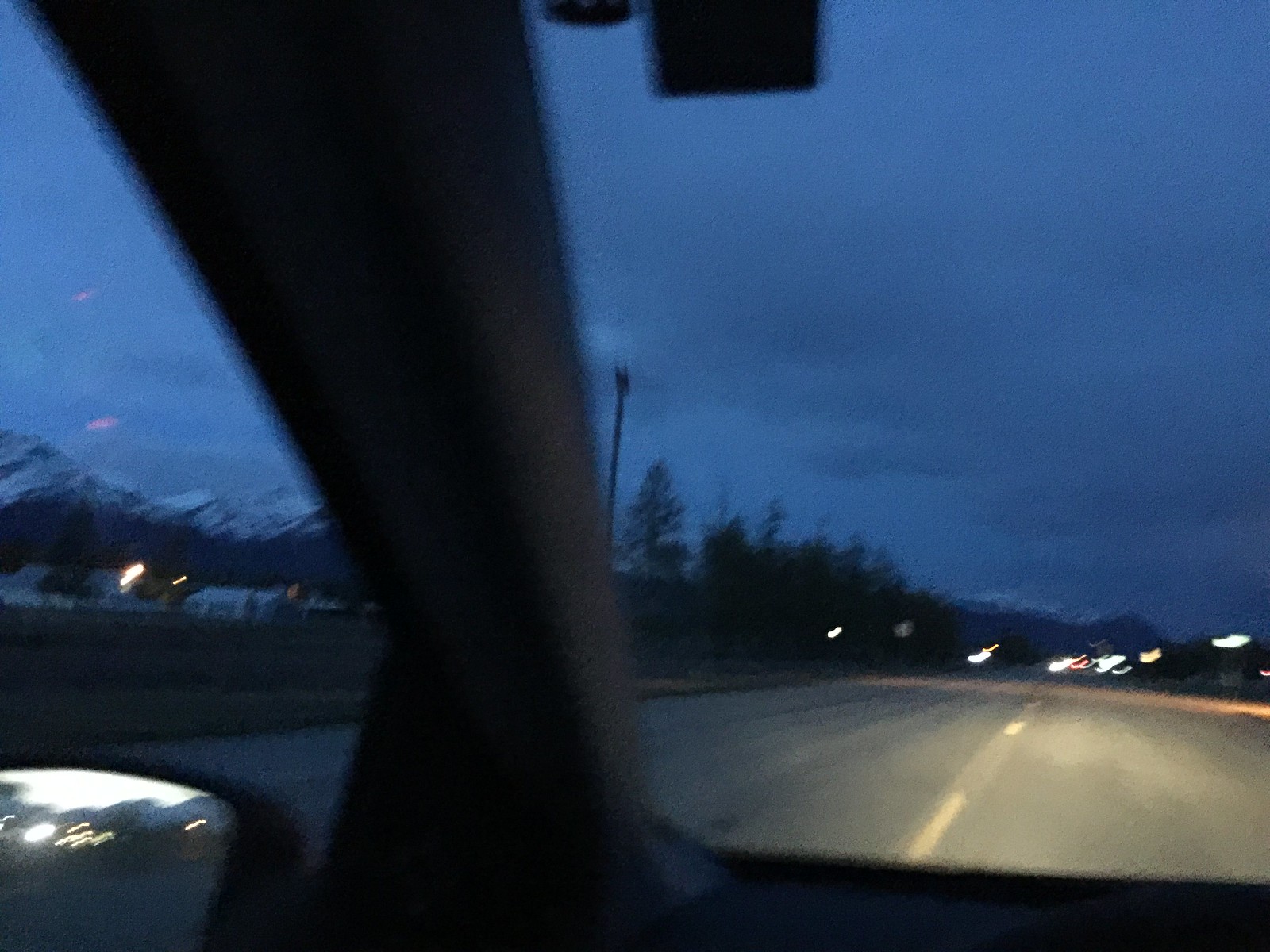A scenic photograph taken from within a moving car, capturing a wide road with a combination of solid and dotted yellow lines running down the middle. Streetlights, possibly mixed with vehicle lights, create a bright trail that seemingly hovers above the center of the road. On the left side, charming houses are nestled against serene, snow-capped mountains under an overcast, gray sky. The landscape is dotted with numerous evergreen trees. The car’s left side mirror prominently features in the frame, showcasing reflections of various lights behind, including a prominent white circular light.